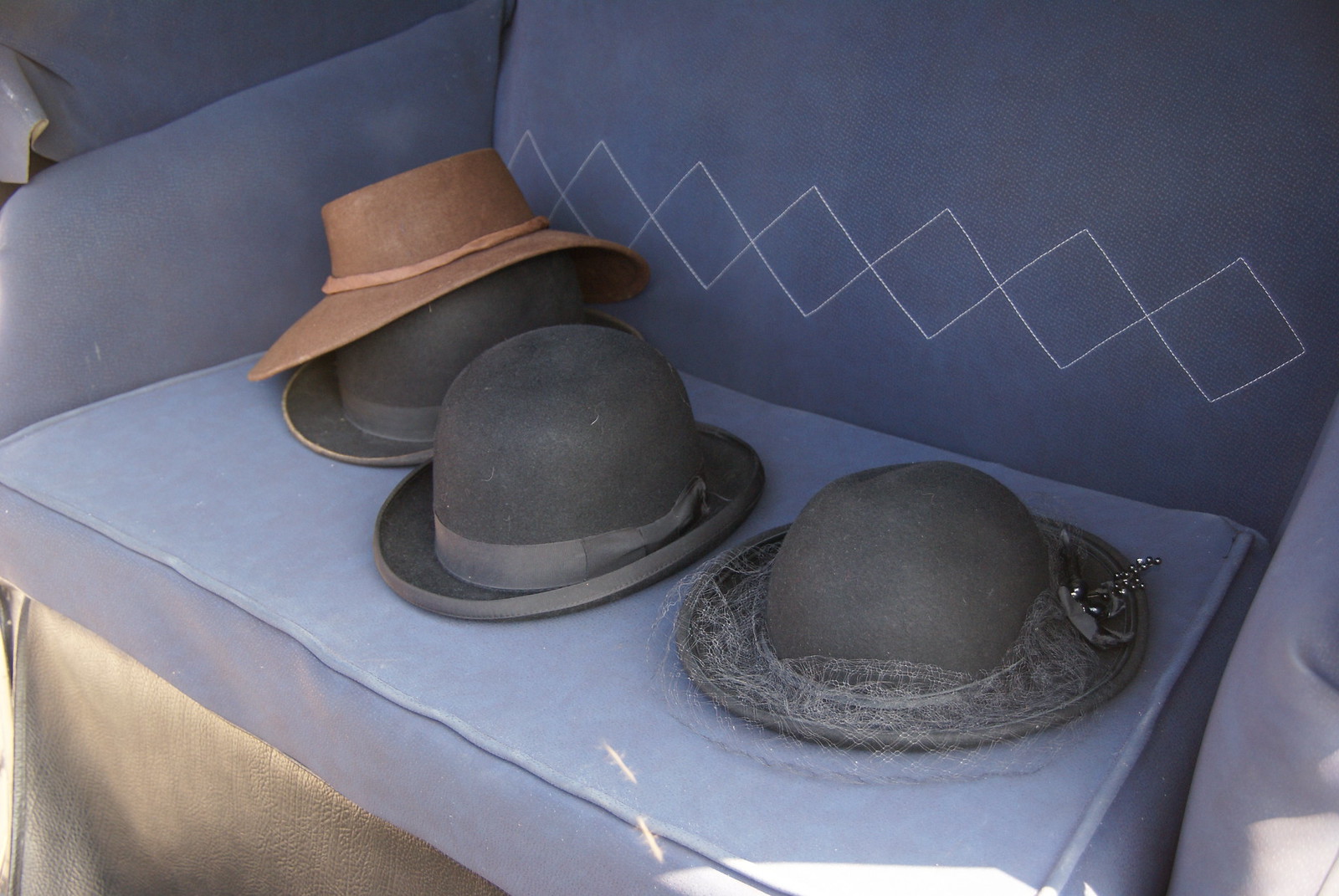A close-up, color photograph showcases a blue leather passenger seat, possibly from a horse-drawn carriage or vintage automobile, suggesting a museum or historical dress-up event setting. Sunlight streams onto part of the seat's front cushion, highlighting intricate details. The cushioned backrest displays a design of diamonds intricately stitched with thin white thread. Positioned on the seat are four hats. On the left side, a gray bowler hat is topped with a brown leather sun hat featuring a loose band and floppy brim. In the center, another men's gray bowler hat with a lighter band sits adjacent to a woman's hat. The latter is gray with lace along the edges, a silvery pin on the right side, and a delicate gray veil netting around the front. Overall, the hats on the blue leather chair provide a glimpse into historical fashion styles.